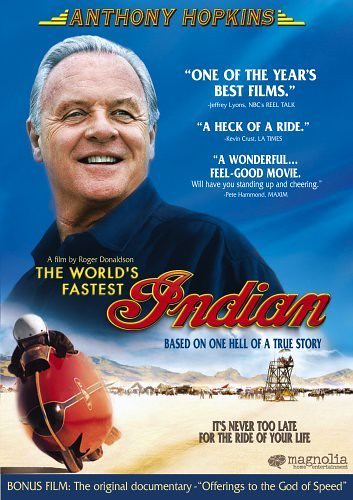The vertical movie poster features a prominent close-up of Anthony Hopkins, smiling and looking to the side, against a two-section background with a blue sky. Above his head, his name "Anthony Hopkins" is centrally displayed with a designed yellow logo on each side. Surrounding his face are glowing reviews: "One of the year's best films" by Jeffrey Likens, NBC Real Talk; "A Heck of a Ride" by Kevin Cruz, LA Times; and "A wonderful feel-good movie, We'll Have You Standing Up and Cheering" by Pete Hammond Maxine. Dominating the center of the poster are yellow and large red bold letters spelling out the movie title "The World's Fastest Indian," along with the caption "based on one hell of a true story" in blue. Below, a desert scene with mountains in the background sets the stage, featuring a red motorcycle driven by a person in a white helmet, surrounded by tents, flags, and spectators. At the bottom left, the text "It's never too late for the ride of your life" appears, alongside the Magnolia Home Entertainment logo. The lower border of the poster in blue includes the text "Bonus film: the original documentary 'Offerings to the God of Speed.'" The overall color scheme prominently integrates blue, yellow, and red.